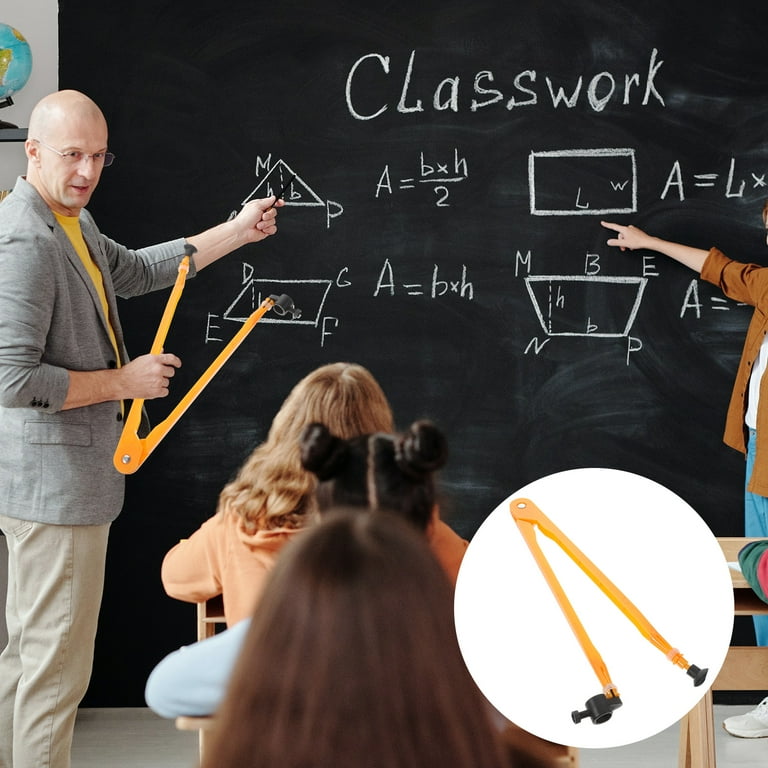The image depicts a horizontal, rectangular classroom scene featuring a teacher and students. At the forefront, a large blackboard takes up the majority of the space, with "Classwork" written in chalk at the top. The board is covered in various geometry equations and shapes, including triangles and other polygons, along with corresponding formulas. 

Standing to the left is a bald, glasses-wearing male teacher dressed in khaki pants, a yellow shirt, and a gray sports jacket. In his right hand, he holds a large V-shaped, yellowish device with black edges, possibly a specialized tool for the board. His left hand features a small black pointer aimed at the chalkboard. On the right-hand side of the photo, partially out of the frame, another individual appears to be pointing at the board.

In the classroom, several students are seated at desks, focusing on the board. Notably, at the bottom right corner of the image, a white circular callout highlights the same V-shaped device the teacher is holding, suggesting it might be the focal point, possibly for an advertisement.

This detailed setup effectively captures a moment of academic instruction, emphasizing the educational atmosphere and the use of geometric tools.